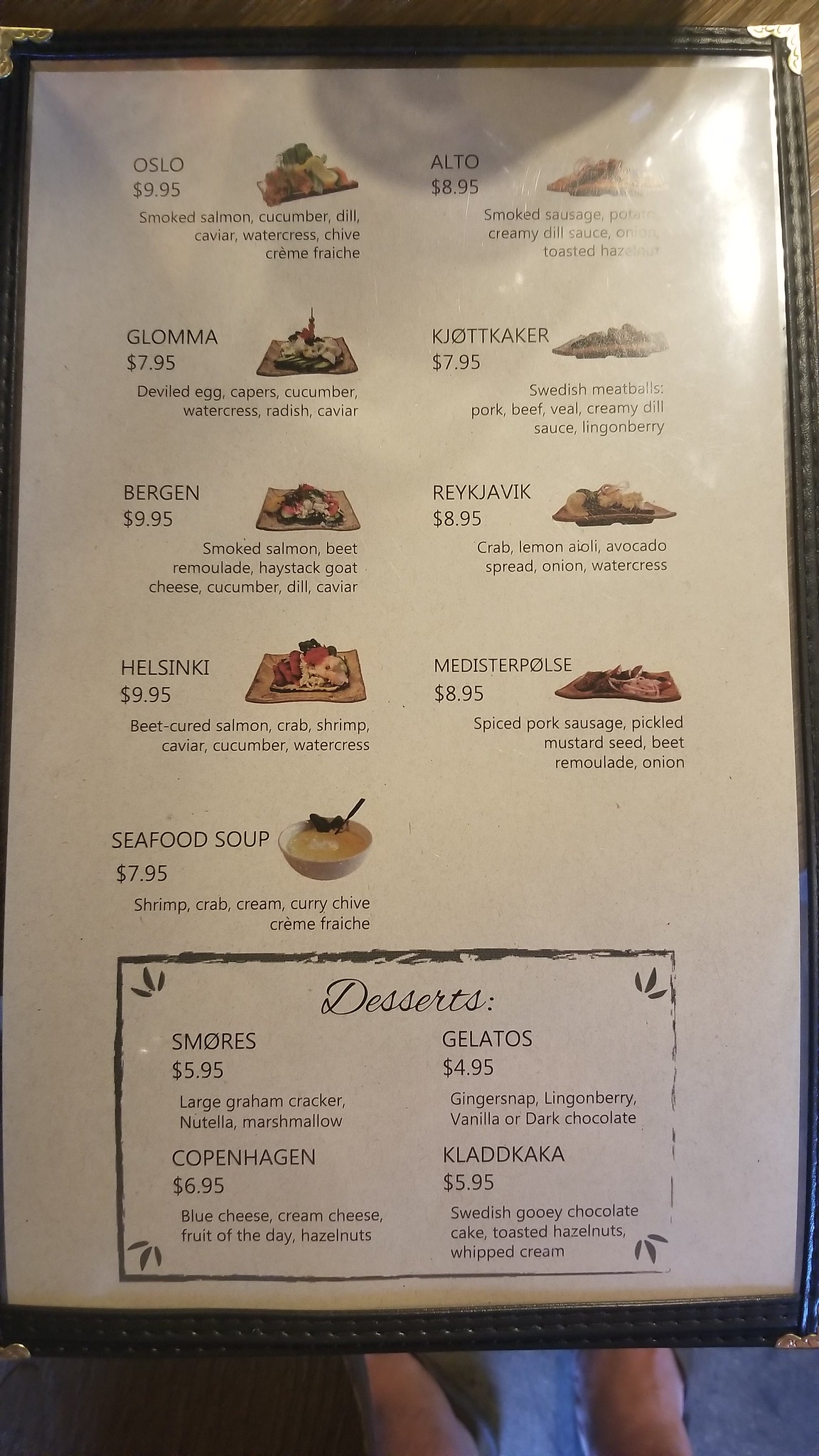This is a detailed and beautifully crafted menu featuring an array of enticing dishes and desserts. The menu is presented on a white background with a striking black border. Each menu item is accompanied by a clear, appetizing image to give a visual representation.

The first item featured is the "Oslo," offered at $9.95, which comprises smoked salmon, cucumber, dill, caviar, watercress, chive, and crème fraîche.

The menu continues with items such as "Alta" and "Gloma," although the specific details for these are not provided in the caption. There is also a dish described in a different language but known as traditional Swedish meatballs. This dish includes a combination of pork, beef, veal, creamy dill sauce, and lingonberry.

Other listed items include "Bergen," "Rye," "Kjavik," and "Helsinki." One particularly detailed dish is "Medestrupulse," which features spiced pork sausage, pickled mustard seed, beet, remoulade, and onion.

Additionally, the menu offers a flavorful seafood soup made with shrimp, crab, cream, curry, chive, and crème fraîche.

At the bottom of the menu, a delightful assortment of desserts is mentioned, such as s'mores, "Copenhagen," gelato, and a rich dessert called "Kladdkaka."

Overall, this menu offers a diverse selection of items, each meticulously detailed to entice diners with both visual and descriptive appeal.